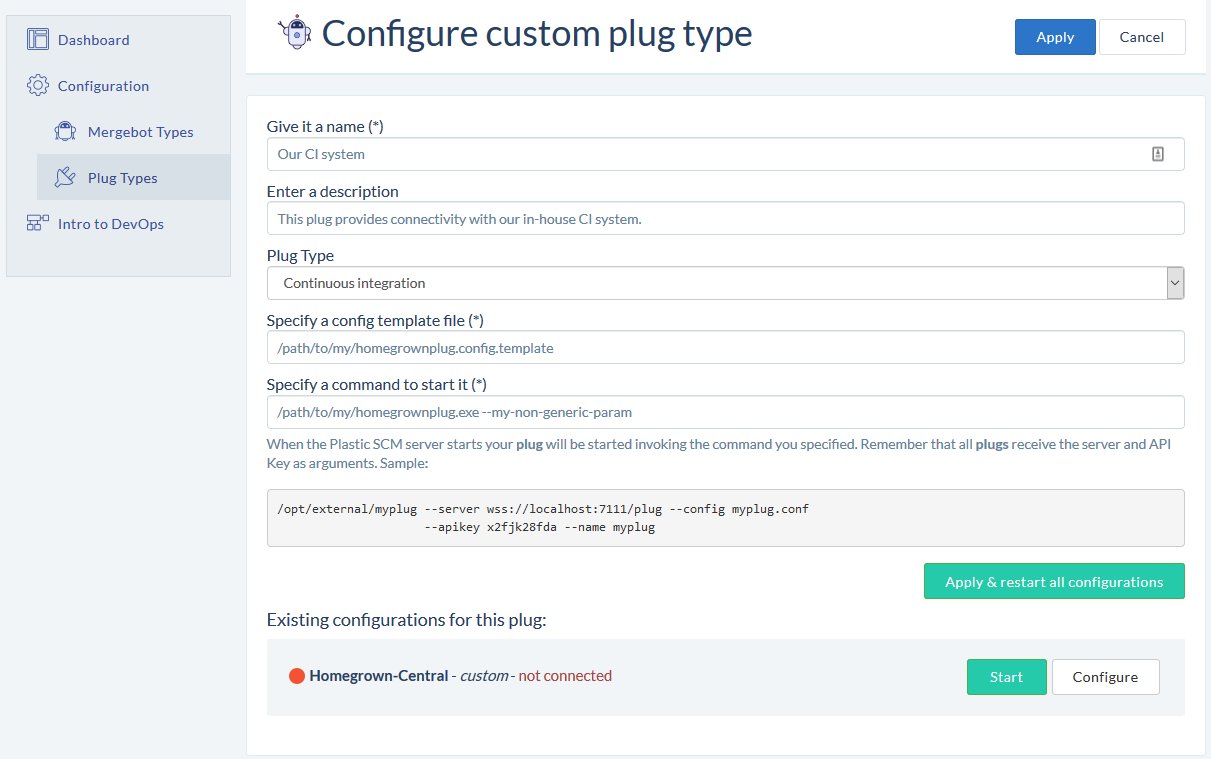This is a detailed screenshot taken from a computer monitor displaying the "Configure Custom Plug Type" window. 

On the left side of the window, a vertical light gray-green banner features several sections. At the top, it reads "Dashboard" next to a square icon. Below that, "Configuration" is displayed in either dark or gray lettering beside a gear icon. Further down, there is an entry labeled "Merge Bot Types" accompanied by a small robot icon on the left. Following that, an electric plug icon precedes the text "Plug Types." Toward the bottom left is a section labeled "Intro to DevOps," symbolized by a diagram of squares.

Centered at the top of the window, a gray cartoon robot man is visible. To the right of this image, in dark lettering, is the heading "Configure Custom Plug Type." Below this heading, a white section contains several text fields and labels. The first field, labeled "Give it a name," is filled in with "Our CI system." Next, a field labeled "Enter a description" reads, "This plug provides connectivity with our in-house CI system." Following this, a field labeled "Plug Type" displays "Continuous Integration."

Further down, there is a section labeled "Specify a config template file" with an asterisk in parentheses, followed by a field containing a directory path structure line. Similarly, another section labeled "Specify a command to start it" also includes an asterisk in parentheses and shows a path statement.

At the bottom of this section, in light bluish-gray lettering, it notes: "When the Plastic SCM service starts, your plug will be started invoking the command you specified." Beneath that, in a gray box with black lettering, a path statement with some configuration information is present.

In the bottom right corner, a long rectangular green button with white lettering reads "Apply and Restart All Configuration." Below this button, to the left, is a green button with white lettering labeled "Start," and to the right, a white button with black lettering labeled "Configure."

In the very lower left-hand corner, the text reads "Homegrown-Central Custom, not connected" in red, accompanied by a red dot to the left.